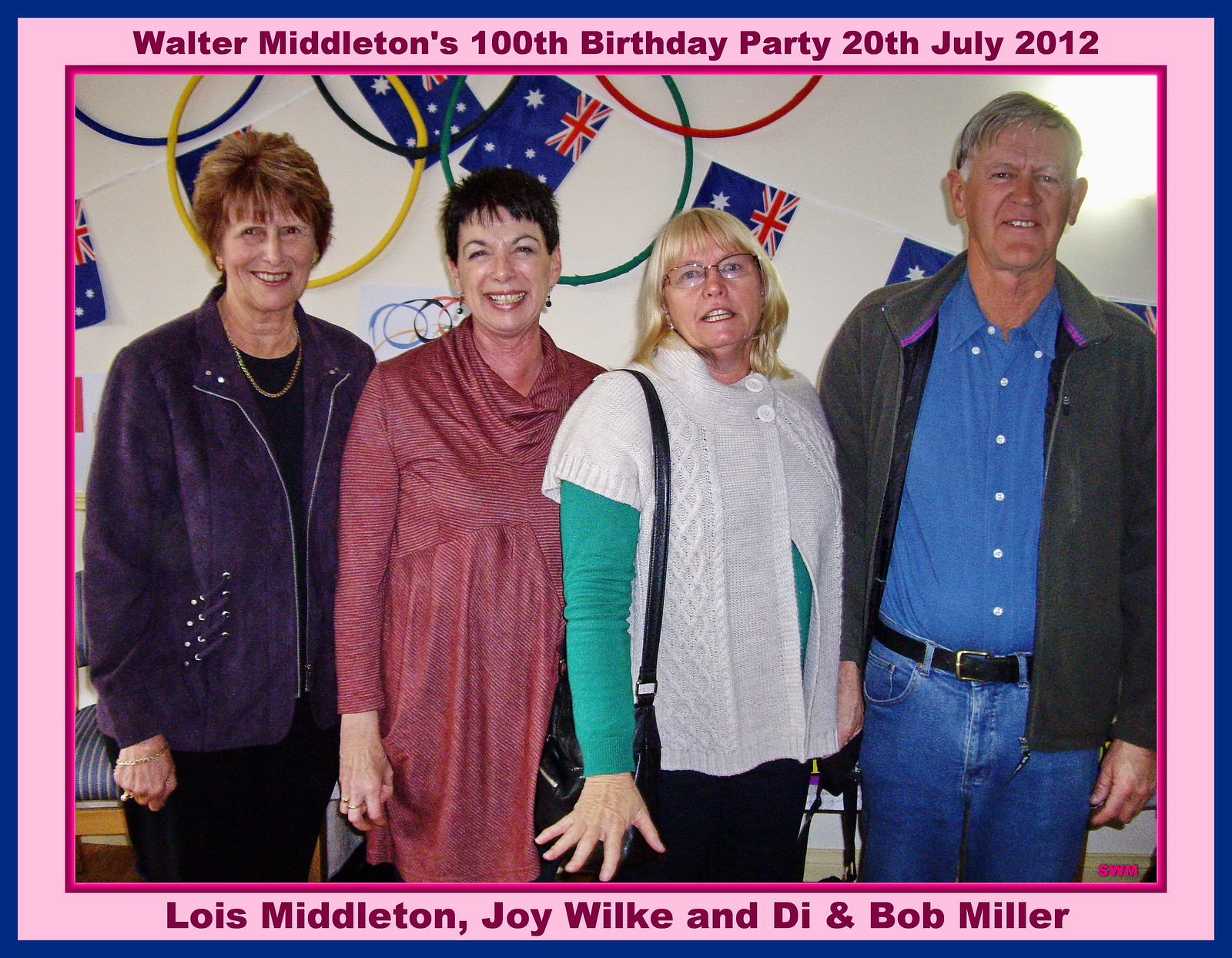In this detailed photograph, four people are standing together at Walter Middleton's 100th birthday party, held on July 20, 2012. The woman on the far left, identified as Lois Middleton, has short red hair, is smiling broadly showing her teeth, and is dressed in a red jacket over a black suit, with a gold necklace adding a touch of elegance. Next to Lois, on her right, is Joy Wilk, who is wearing a light purple dress and also smiling with her teeth visible, her eyes slightly squinted, and her hand resting on her hip with fingers curled in. To Joy's right stands Dee Miller, the shortest in the group, with blonde hair and glasses. She is dressed in a green long-sleeved shirt layered under a white sweater, her hands hanging down with fingers spread wide open. The gentleman on the far right, Bob Miller, has gray hair parted to the right and is wearing a blue shirt under a gray jacket, paired with blue jeans. A pink border surrounds the photograph, and there is a banner in the background decorated with British flags. Beneath the image, the caption provides the event details and the names of the individuals: Lois Middleton, Joy Wilk, and Dee and Bob Miller.